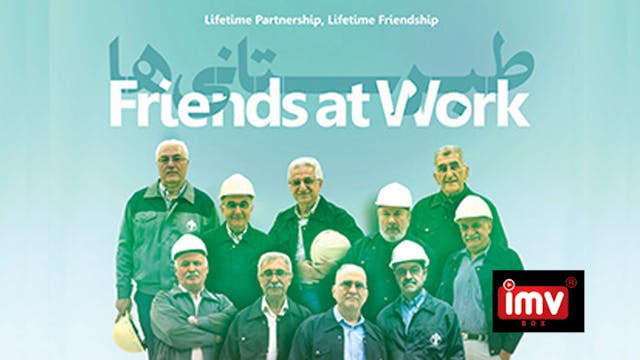This image appears to be an advertisement or a public service announcement with a faded gradient background transitioning from light green at the top to pale blue at the bottom. Centered at the top in small white letters, it reads "Lifetime Partnership, Lifetime Friendship." Just below, in larger white letters, it says "Friends at Work," with the same phrase also appearing in Arabic interwoven between the English words. The image features 10 senior gentlemen, likely in their 60s, all smiling and demonstrating camaraderie. They are arranged in two levels, with five men standing behind five others. Half of the men are wearing construction helmets, while the others hold their helmets – one man holding his by his side and another crossing it over his chest. Each of them is wearing zip-up jackets, and several of the men sport mustaches, with one having a beard, and nearly half wearing glasses. Superimposed towards the bottom right of the image is a black square containing a smaller red square with the white lowercase initials "IMV." The overall scene communicates a theme of long-standing friendship and partnership in a construction-related setting.